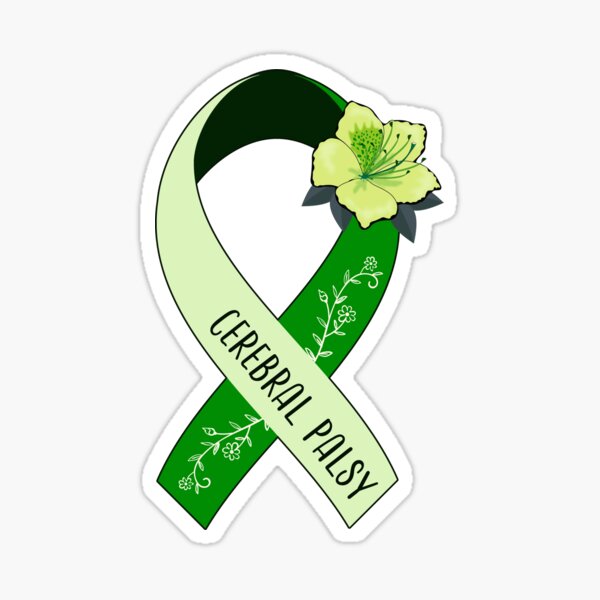The image features a green awareness ribbon prominently displayed on a white background. The ribbon, which could be perceived as a sticker, consists of two shades of green: the left side is light green, while the right side is darker green. The darker side is adorned with intricate white floral stenciling, and near the top right of this side, there is a distinctive green flower with gray leaves, symbolizing cerebral palsy awareness. The light green side of the ribbon bears the text "CEREBRAL PALSY" written in bold, black, capital letters. The entirety of the ribbon is outlined in a thin gray line, enhancing its visibility against the plain backdrop. The ribbon's loop formation creates a figure-eight-like shape, lending a simple yet meaningful visual impact to the design.